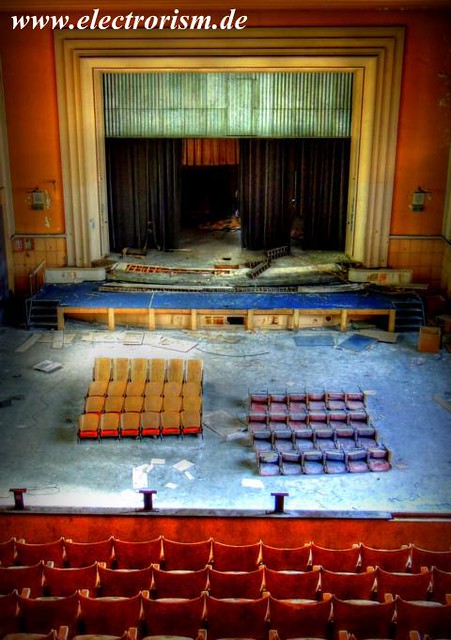The photograph captures the view from the balcony of an old, decaying theater. The vantage point looks down towards the empty stage with its blue backdrop and black curtains. The once-grand theater shows significant signs of disrepair. The first floor seating is largely absent, with only a few red chairs remaining amidst concrete and dust, suggesting a space under renovation or deconstruction. Some sections of disconnected theater seats lie haphazardly on the ground. The stage is cluttered, with exposed wood framing, dirt, and debris scattered across it. The side walls, painted an orangish-coral color, feature light fixtures, and a golden, picture-frame-like structure outlines the stage. At the top left corner of the photograph, the text www.electroism.de is displayed, marking the image.